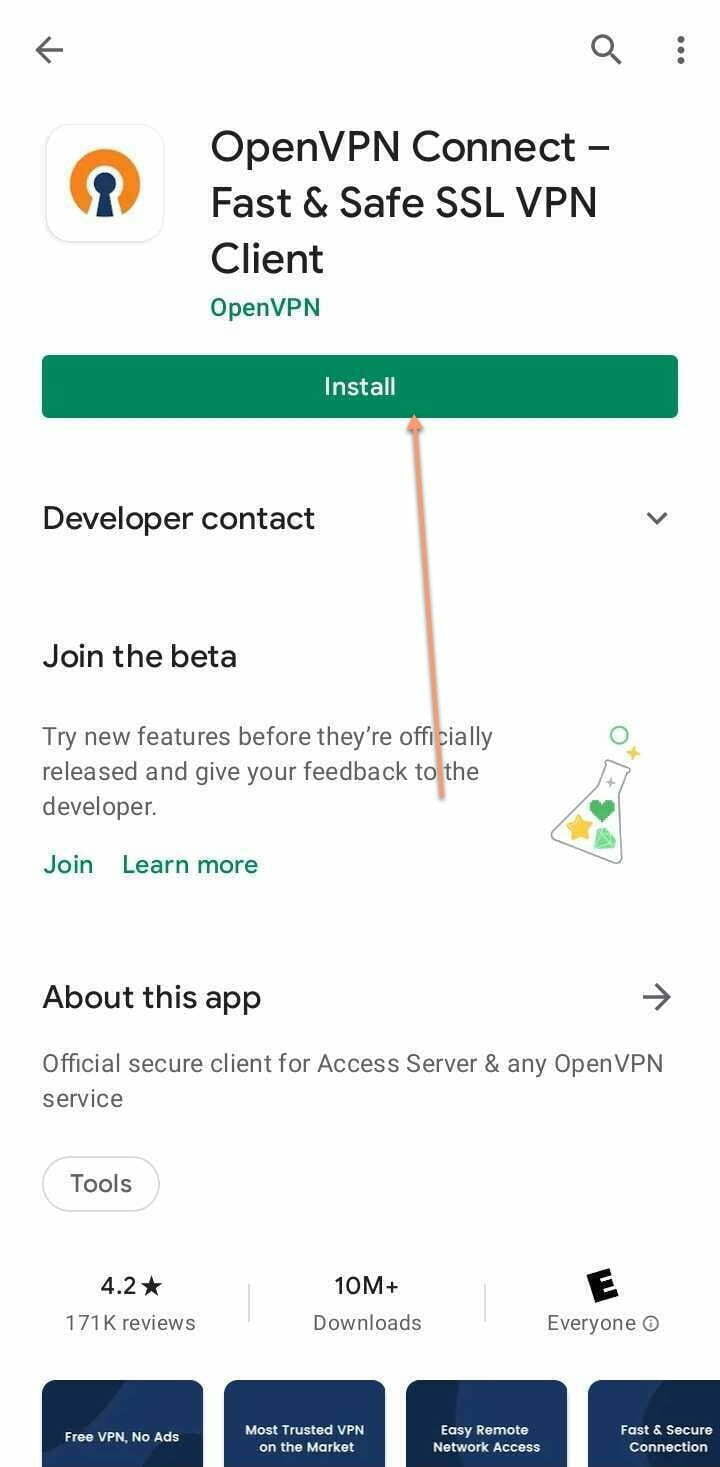**Detailed Caption:**
The image depicts a product page for the "OpenVPN Connect" application, which is described as a fast and safe SSL VPN client. At the top of the page, there is a back arrow for navigation. The app's icon is prominently shown on the left; it features a white box with an orange and blue design resembling a keyhole lock, with the orange outline forming the outer part of the lock.

Below the app icon, there's a teal "Install" button with white text centered on it. An orange user-imposed arrow points leftward, positioned to the left of the install button. Further down, there is the "Developer Contact" section, accompanied by an arrow indicating that this option has not been selected yet.

Beneath that, the page invites users to "Join the Beta" program, encouraging them to try new features before their official release and provide feedback. This section includes a "Join & Learn More" button and an icon resembling an Erlenmeyer flask filled with a yellow star, a green heart, and a blue diamond.

The "About this app" segment follows on the right, stating that it is the official secure client for Access Server and any OpenVPN service. The app is categorized under "Tools," indicated by a grayed-out box. Lastly, the page has sections for reviews, downloads, and information on the app's suitability for all users, accompanied by four small icons.